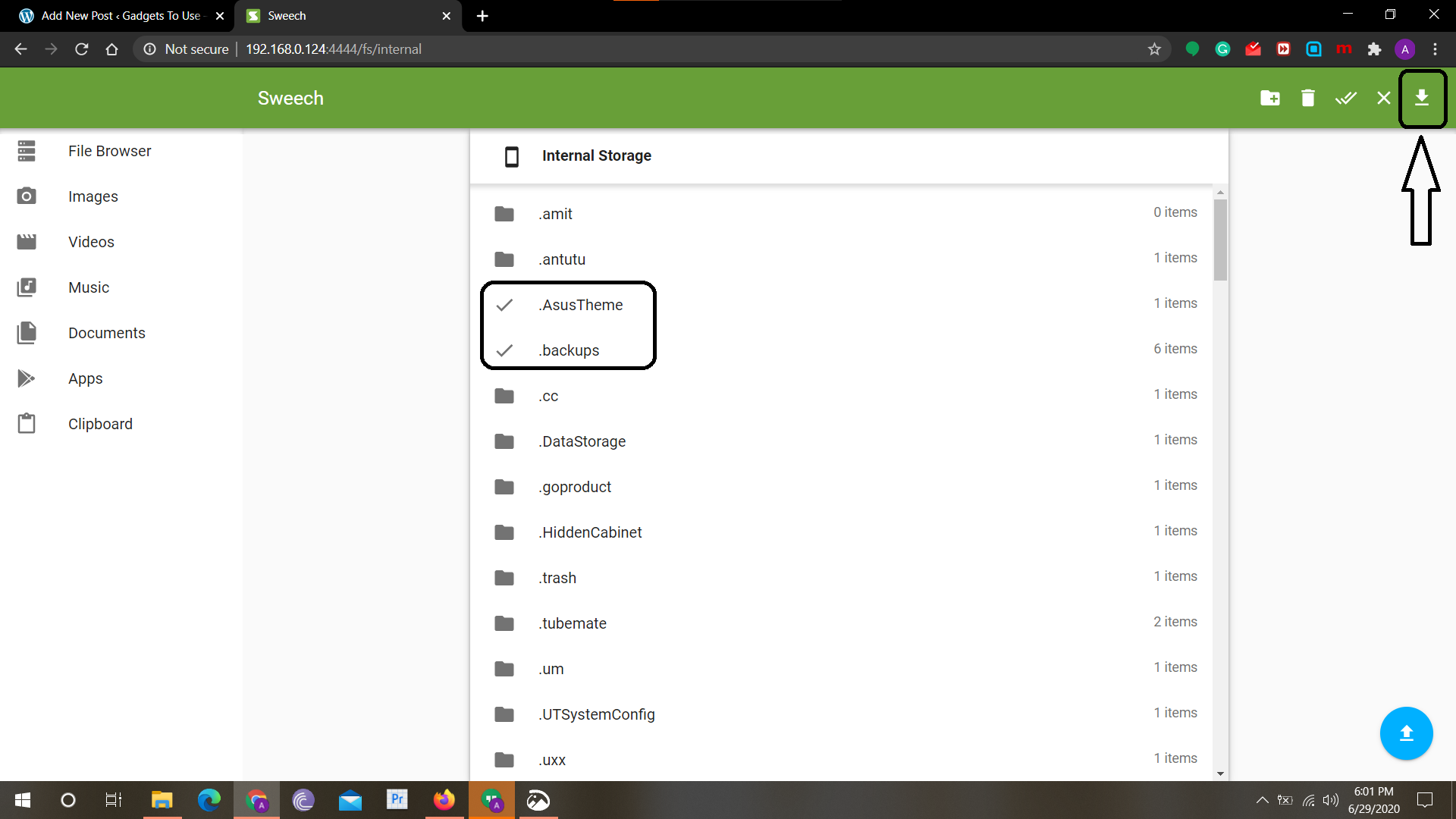This is a detailed desktop screenshot of the Switch app, a file transfer utility designed for Android devices to facilitate the transfer of files from a smartphone to a computer. Dominating the top of the screen, a large green banner is prominently displayed, with the word "Switch" positioned towards the left in small white letters. Adjacent to this banner on the right is a row of functional icons including folder, trash, checkmarks, an X, and a download symbol. 

The download icon is distinctly highlighted with a black box around it, further emphasized by an edited white arrow pointing directly at the download box, drawing attention to its purpose. Below this row, under the section titled "Internal Storage," two particular options are highlighted with a black box: "ACES theme" and "Backups."

The marked boxes and icons suggest a step-by-step instructional guide. It appears that the user is directed to click on the "ACES theme" and "Backups" options under "Internal Storage" and then use the download button to transfer these selected files to the computer. The screenshot seems to serve an educational or tutorial purpose, effectively guiding the user through the process of downloading files from their Android device using the Switch app.